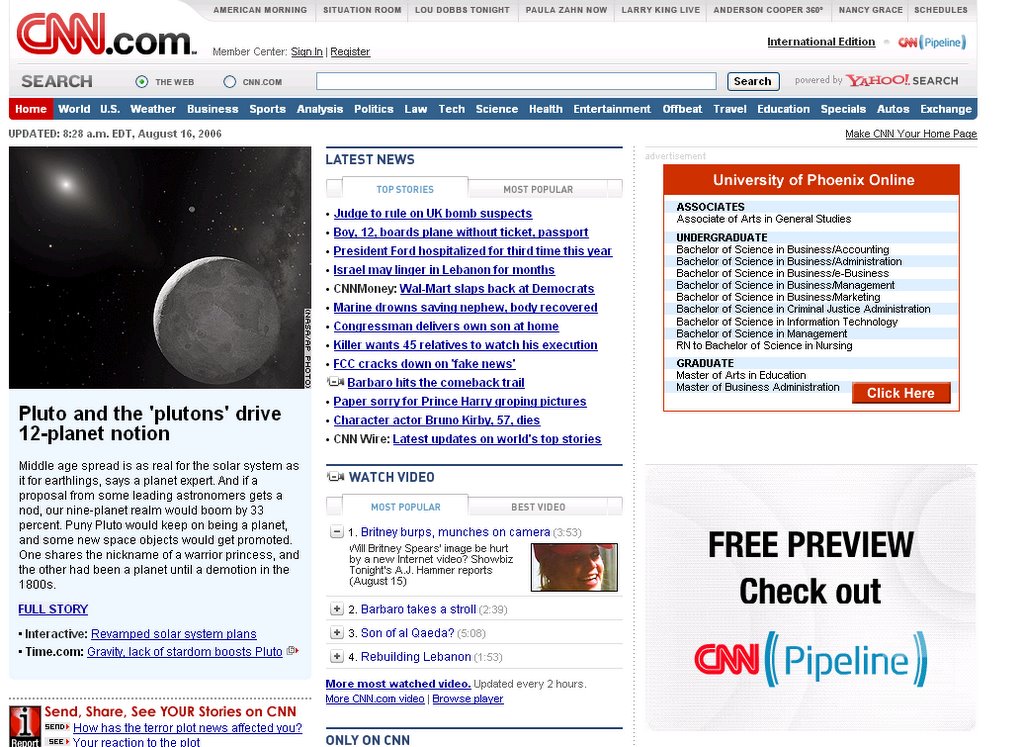This screenshot captures the homepage of the CNN.com website. In the upper left-hand corner, the "CNN.com" logo is prominently displayed. At the very top are eight navigation tabs: American Morning, Situation Room, UDOPS Tonight, Paula's On Now, Very Clean Live, Anderson Cooper 360, Nancy Grace, and Schedules. Adjacent to these are links to the Member Center, Sign-in/Register, International Edition, and CNN Pipeline. Just below, a search bar powered by Yahoo Search allows users to search either the web or CNN.com.

Directly beneath the search bar are several navigation tabs: Home, World, U.S., Weather, Business, Sports, Analysis, Politics, Law, Tech, Science, Health, Entertainment, Offbeat, Travel, Education, Specials, Autos, and Exchange. Additionally, there is an option to make CNN your homepage.

On the left side of the page, it is indicated that the content was updated at 28 a.m. EBT, which translates to August 16, 2016, in Eastern Standard Time. A notable featured image shows a dark night sky with the sun illuminating what appears to be Pluto. The caption below the image reads, "Pluto and the Plutons Drive 12 Planet Notion," elaborating that the image indeed depicts Pluto. A small introductory paragraph about the story is provided with a link to read the full article.

To the right of the main feature, the latest news section includes several items such as "Paper Sorry for Prince Harry Pictures" and "President Ford Hospitalized for Third Time This Year." There is also a "Most Popular" section and options to watch videos. Among the most popular videos, the top one is titled, "Britney Burps Munches on Camera."